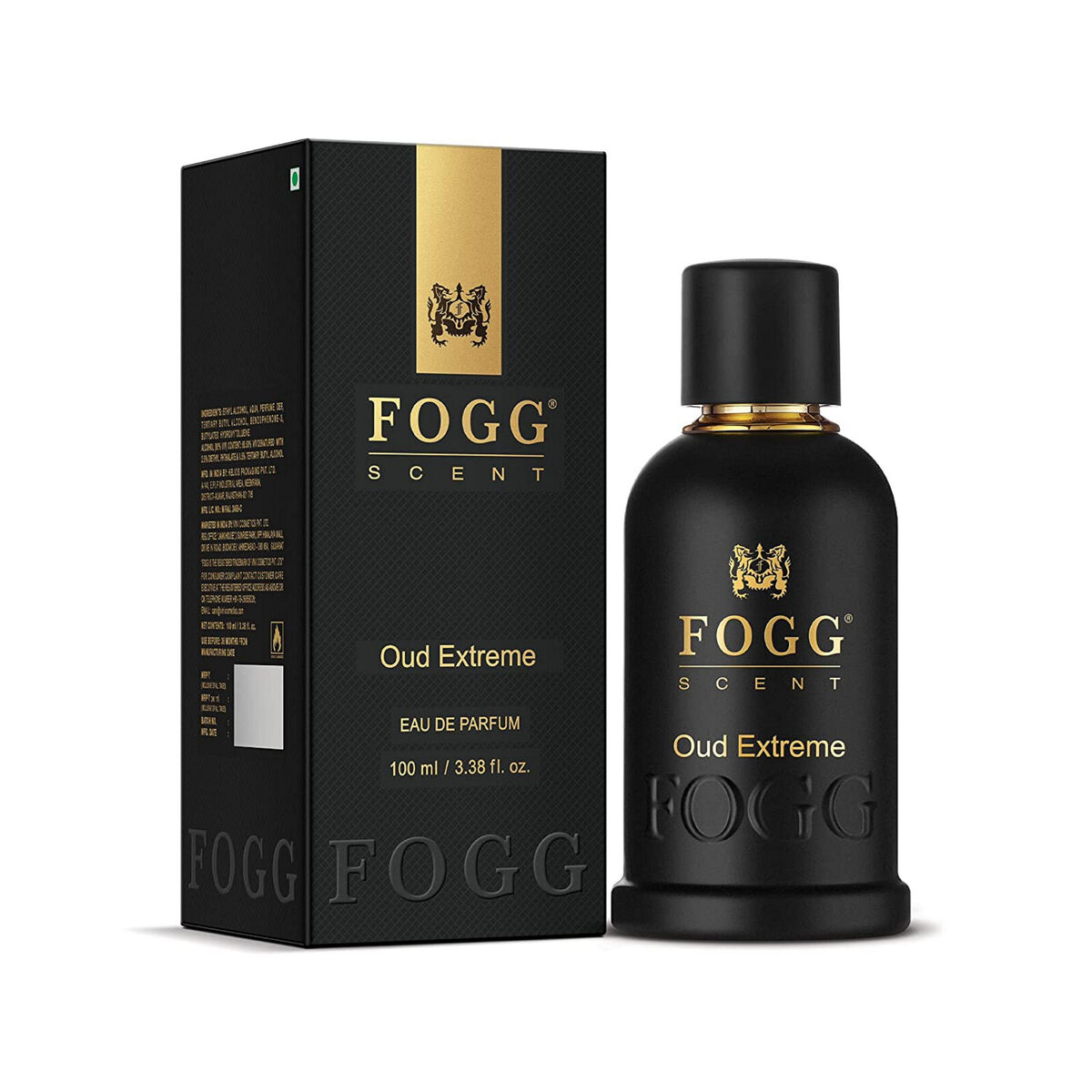A high-quality colored photograph showcases a sleek, luxurious cologne designed to captivate attention. The product, a sophisticated Fog Scent cologne, is meticulously arranged against a pristine white background—emphasizing its elegance as the sole item in the image. Positioned strategically, the bottle and box are side by side, with the box on the left and the cylindrical bottle on the right.

The box, shown in a three-quarter view, is adorned with an eye-catching logo featuring two golden horses and a crest at the front, prominently displaying the brand name "Fog Scent" in gold lettering. Below, the words "Oud Extreme" can be found. Additional product information adorns the sides and back of the box, indicating it contains a 100ml (3.38 fluid ounces) Oud De Parfum.

The bottle itself is a study in minimalist sophistication—a matte black cylinder standing slightly shorter than the box, approximately four inches in height. It mirrors the box's branding, complete with the gold-embossed logo and the labels "Fog Scent" and "Oud Extreme." The black cap, topped with a shiny gold rim, completes the lavish presentation, making it clear that this product is designed for those with refined tastes.